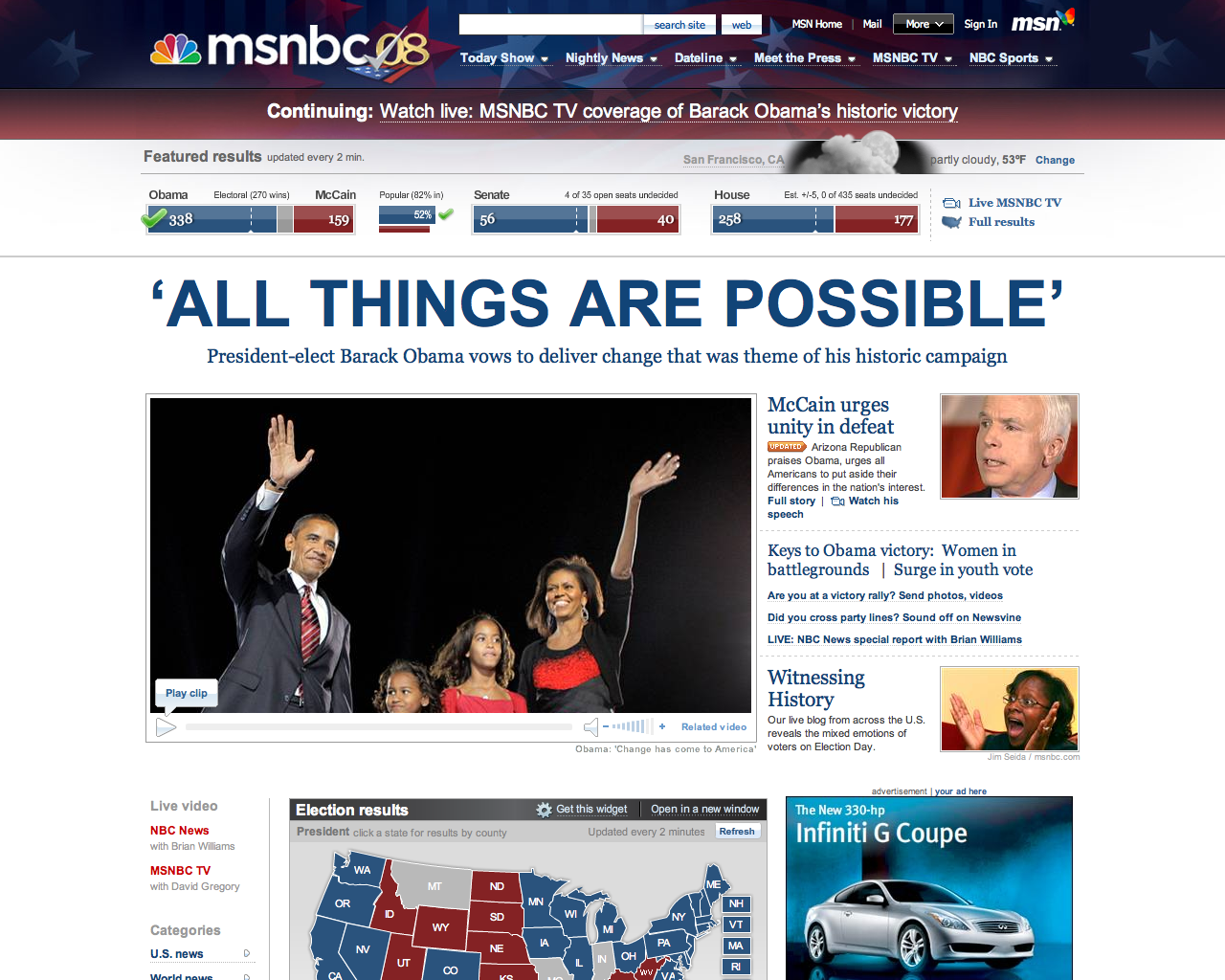This image is a detailed screenshot taken from the MSNBC webpage, specifically archived from the 2008 election. The layout is predominantly a large square format.

To the right of the main content, there is a search bar followed by a web button. Adjacent to this are options labeled MSN Home, Mail, and a drop-down menu that says 'More'. There is a button for sign-in next to the MSN logo.

Beneath this header, there is a navigation bar with tabs titled Today Show, Nightly News, Dateline, Meet the Press, MSNBC TV, and NBC Sports. Each tab includes drop-down options. The background for this row is designed to mimic the American flag, rendered in a contemporary, wavy style of stars and stripes.

Directly below the navigation, a red banner announces: "Continuing Watch Live MSNBC TV coverage of Barack Obama's historic victory." Below this banner, it indicates, "Feature results updated every two minutes." The sidebar provides local weather information for San Francisco, California, reporting partly cloudy skies and a temperature of 53°F.

The screenshot captures a historic moment, highlighting Barack Obama's electoral victory with 338 electoral votes to John McCain's 159, along with Obama receiving 52% of the popular vote. It displays results reflecting the Democrats winning 56 Senate seats to the Republicans' 40, and 258 House seats to the Republicans' 177.

At the bottom, a blue text header reads, "All Things Are Possible," accompanied by a quote from President-elect Barack Obama, vowing to bring about the change that was the theme of his historic campaign.